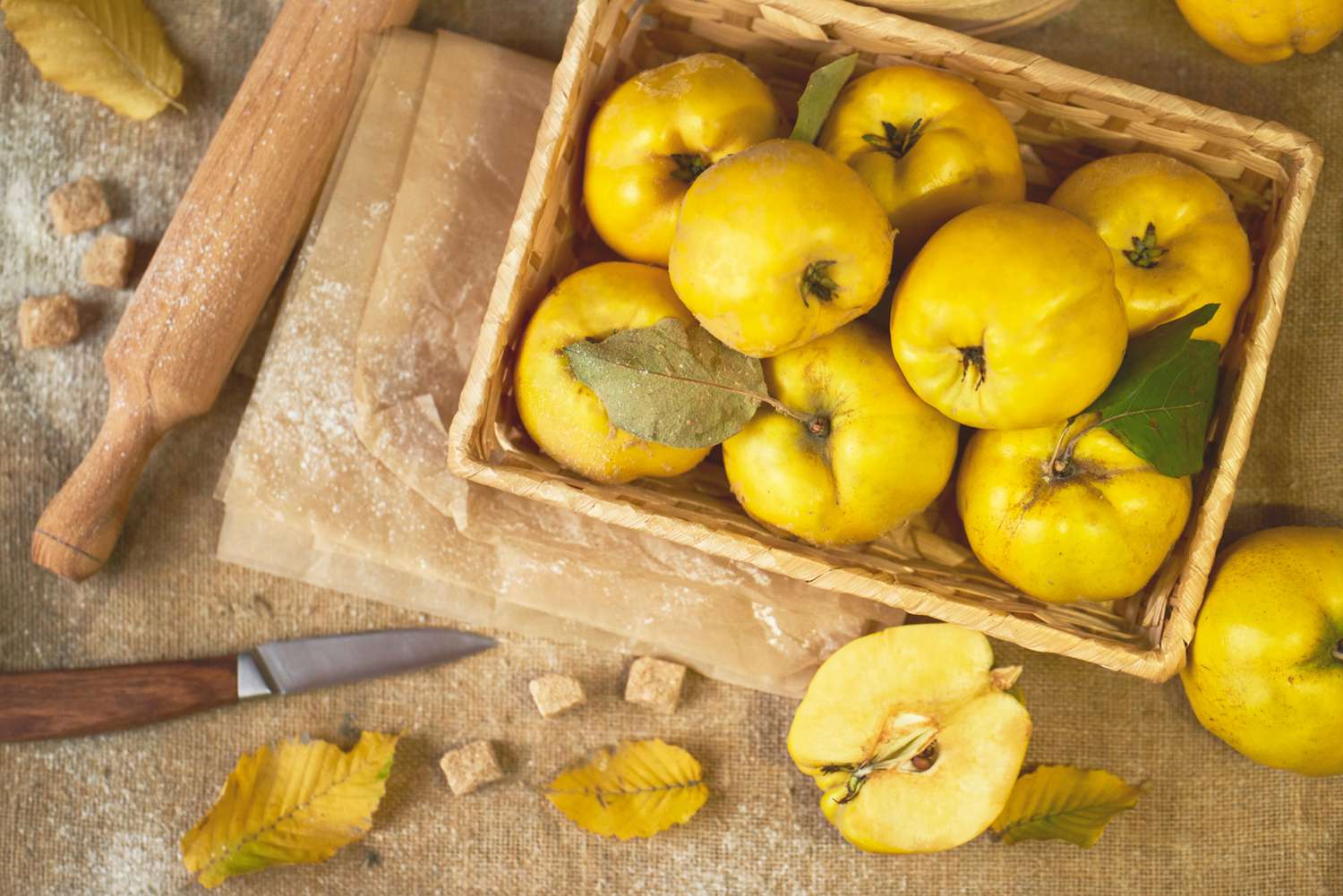In this detailed, overhead photograph, we see a rustic tableau of aged golden granny apples, clustered in a woven wooden basket, showcasing their pale to medium golden hues. One of these apples, cut in half and positioned at the bottom center-right outside the basket, reveals its seeds still intact, indicating it was sliced a few hours ago. Stems are absent from the apples, noting their age. A small butter knife with a wooden handle rests in the bottom left corner, presumably used for slicing. Accompanying this are a rolling pin in the top left sprinkled with a fine white powder, likely icing sugar, which also dusts the hessian cloth-covered table. Some yellow-green leaves, four in total, are scattered strategically among the apples and the scene, along with sugar cubes. Baking parchment lies behind the basket, further dusted with sugar, enhancing the impression that these apples are set for a culinary adventure, perhaps pie or tart-making. The central focus is the basket with its apples, flanked by the rolling pin and knife, woven into a narrative of homely, autumnal baking.